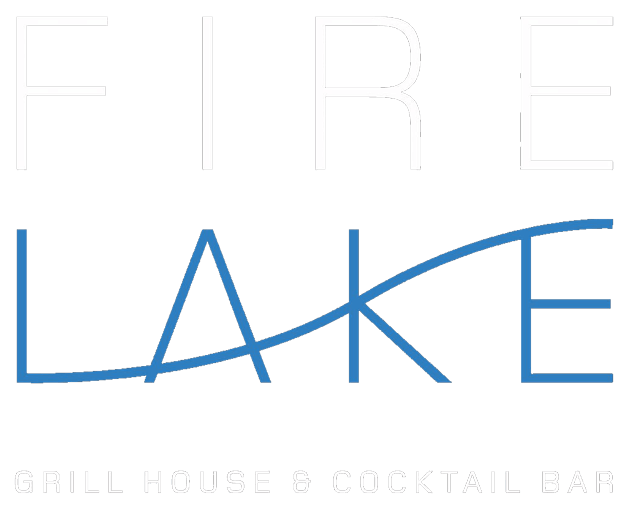This image features a minimalist, stylized logo for the "Fire Lake Grill House and Cocktail Bar." The logo is set against a solid white background. At the top, the word "FIRE" is displayed in faint white capital letters with a thin black outline. Directly below, the word "LAKE" is presented in bright blue text, with a uniquely stylized design where the "L" extends upwards to form part of the "A," the "K," and the "E," resembling a rising hill. Beneath this, the phrase "GRILL HOUSE AND COCKTAIL BAR" is written in smaller, white capital letters with a thin black outline, spread horizontally across the bottom of the image. The entire composition uses only three colors: white, black, and blue, emphasizing the sleek and modern aesthetic of the logo.